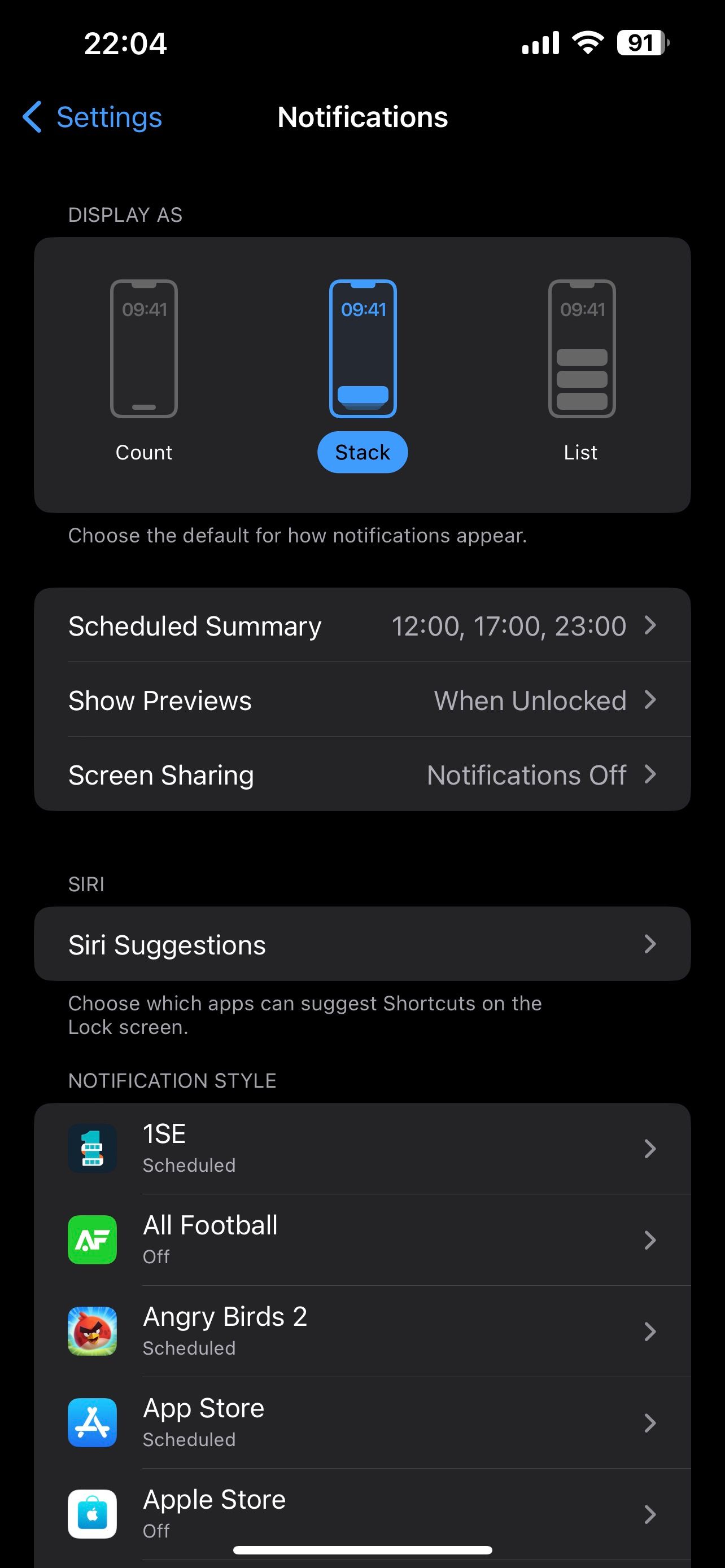The image displays a smartphone screen with various settings and options. In the upper left corner, the time "22:04:04" is shown, alongside network indicators that reveal 4 bars of Internet connectivity and full WiFi signal. The battery icon indicates a 91% charge. 

In the top section, there is a left arrow next to the word "Settings" in blue, and the central heading "Notifications" is bolded in white. Below this, "Display As" appears in grey letters. A grey box presents three different notification display options. The first option is "Count," followed by "Stack," which is highlighted in blue with a blue illustrated phone icon, surrounded by an oblong blue box. The final option is "List" with a grey phone icon over the word "List."

Below these options, it says "Choose the default for how notifications appear." Further down, there is another grey section. It begins with "Scheduled Summary" in white, listing the times "12:00," "17:00," and "23:00," separated by a grey line. The next setting, "Show Previews," states "When Unlocked" with an arrow pointing to the right.

The screen's interface is visually structured to guide the user through accessible settings and customization options.